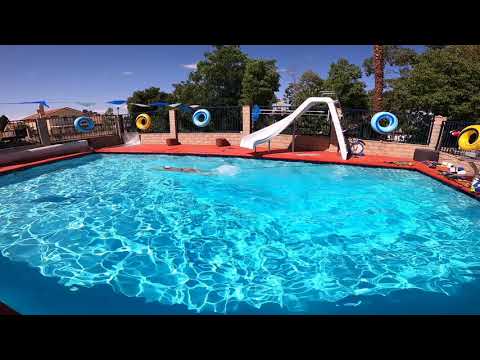In this richly detailed photograph, a vibrant blue swimming pool takes center stage, its water gleaming under the midday sun, producing multiple shiny reflections. The pool features light blue lines, enhancing its bright appearance, and is framed by a red edge accented with a white stripe on the far side. Surrounding the pool is a brown wall topped with a sturdy black fence, adorned with numerous blue and yellow pool toys or floats. A pool slide whimsically curls beside the pool, awaiting eager swimmers. The scene is set against a serene backdrop of lush green trees and a clear blue sky dotted with a few white clouds. This setting, which seems to resemble a community pool in an upscale neighborhood, also hints at a laid-back, possibly Californian atmosphere, complete with a palm tree adding to the ambiance. Two black rectangular bars frame the top and bottom of the image, adding a cinematic quality to the peaceful, sunny day tableau.